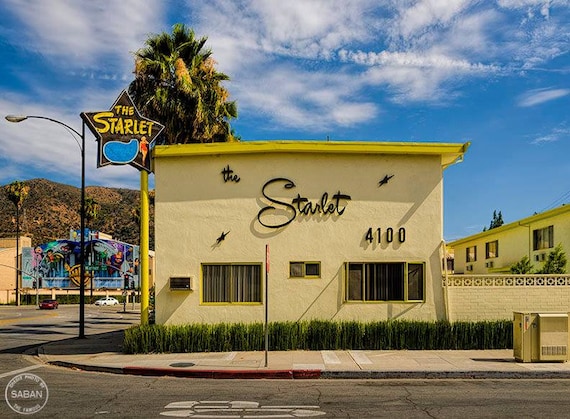In the photo, there is a small, modest yellow building named "The Starlet," identifiable by the black text on its exterior and a matching sign to the left featuring a drawing of a movie star. The Starlet's address number, 4100, is visible on the front, which sports a 50s era cursive sign and is adorned with stars. The building appears to be a two-story hotel or motel situated on a city street, possibly in Los Angeles or Hollywood, given its summery atmosphere and the Hollywood Hills in the background. A large tree stands behind the sign, and the scene includes a red curb, a partial stop sign on the road, and two parked cars - one red and one white. The lower left corner of the image has the watermark "Saban." The building features brown curtain-adorned windows, air conditioner vents, and is accompanied by a brick wall that extends to rooms on the side in the same yellow color. Additionally, there is a star-shaped sign illustrating a woman in a red swimsuit by a swimming pool. In the background, a colorful building with artistic graffiti can be seen, resembling the Warner Brothers symbol. The sky is a bright blue filled with white puffy clouds, completing the vibrant, sunlit scene.